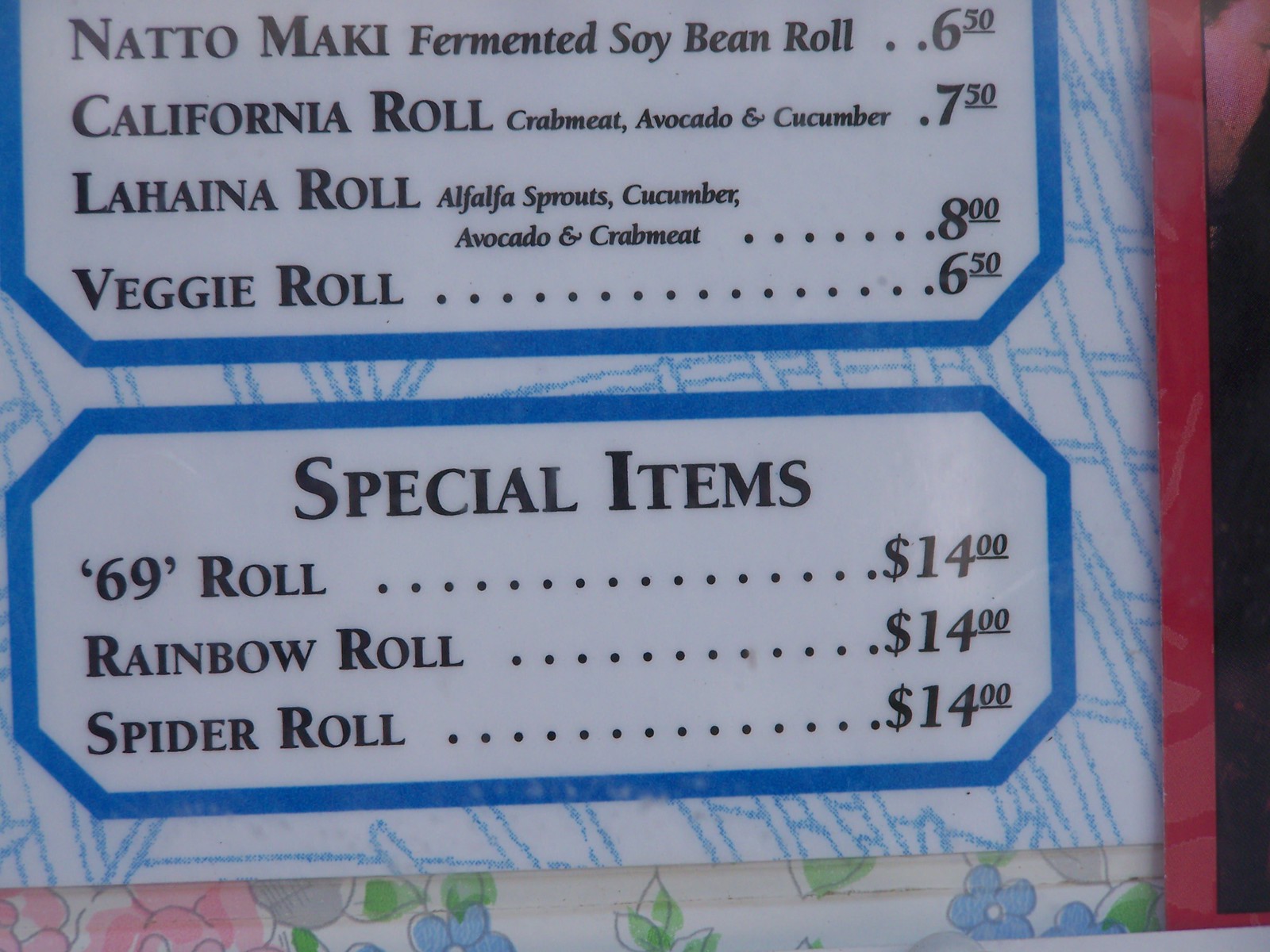This close-up rectangular image shows part of a menu from what seems to be an Asian or sushi-themed restaurant. The menu is mounted on a wall decorated with floral wallpaper, visible beneath it, and bordered on the right side by a red piece of wood. The menu features a vibrant blue and white background with categories outlined in blue. It includes items like "Natto Maki (Fermented Soybean)" priced at $6.50, "California Roll (Crab Meat, Avocado, and Cucumber)" at $7.50, "The Heiner Roll (Alfalfa Sprouts, Cucumber, Avocado, and Crab Meat)" for $8, and a "Veggie Roll" for $6.50. A section labeled "Special Items" lists a "69 Roll," "Rainbow Roll," and "Spider Roll," each priced at $14. The bottom of the menu also features a decorative border of sketched flowers in pink, blue, and green. The predominant colors in the image are the vibrant blue of the menu and the details that accompany it.